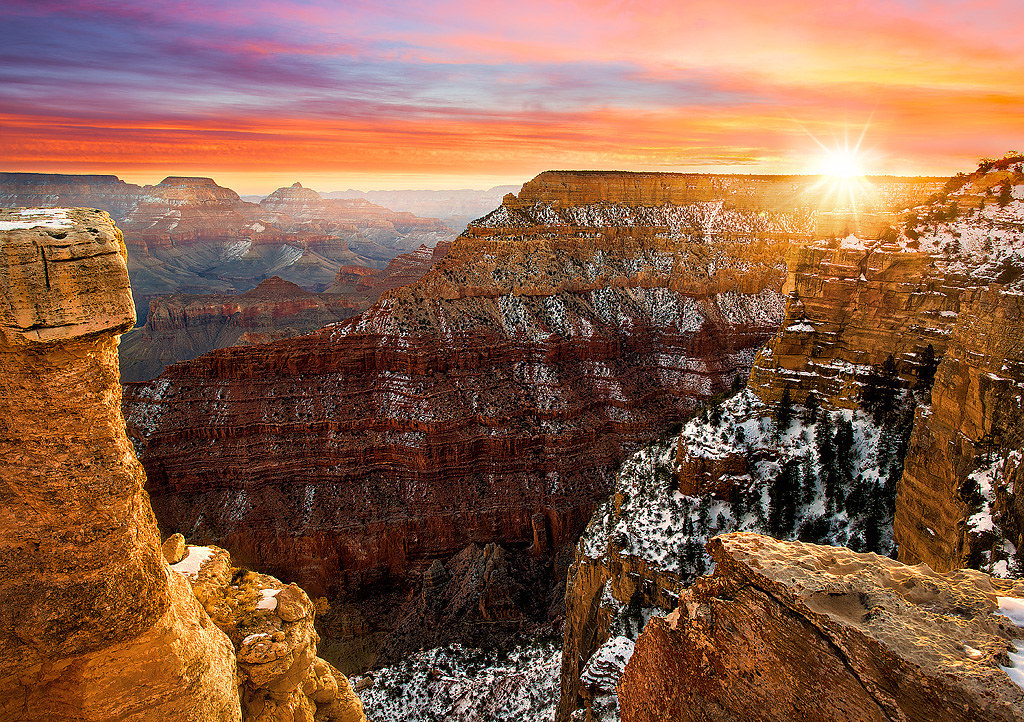This stunning photograph captures an elevated view of the Grand Canyon at sunset, taken from a high vantage point on the side of a mountain. In the bottom left corner, jagged rocks are visible, adding depth and perspective to the composition. To the right, another serrated mountain, blanketed in snow, stands prominently. Dark green fir-like trees populate the snow-covered cliffs and various parts of the mountainous landscape. The left side features a unique, tower-shaped rock formation, resembling the top of a glass bottle. In the expansive background, multiple canyon mountain ranges extend far into the distance, enveloped in a soft mist. The foreground's rugged, brownish-orange rocks with patches of snow and foliage contrast with the distant, fog-shrouded peaks. The sky above is a breathtaking mix of hues—orange, pink, yellow, and hints of blue—reflecting the setting sun whose beams peek from behind one of the distant peaks. The combination of rocky, textured formations, snow, trees, and the myriad colors in the sky creates a visually captivating and serene scene.